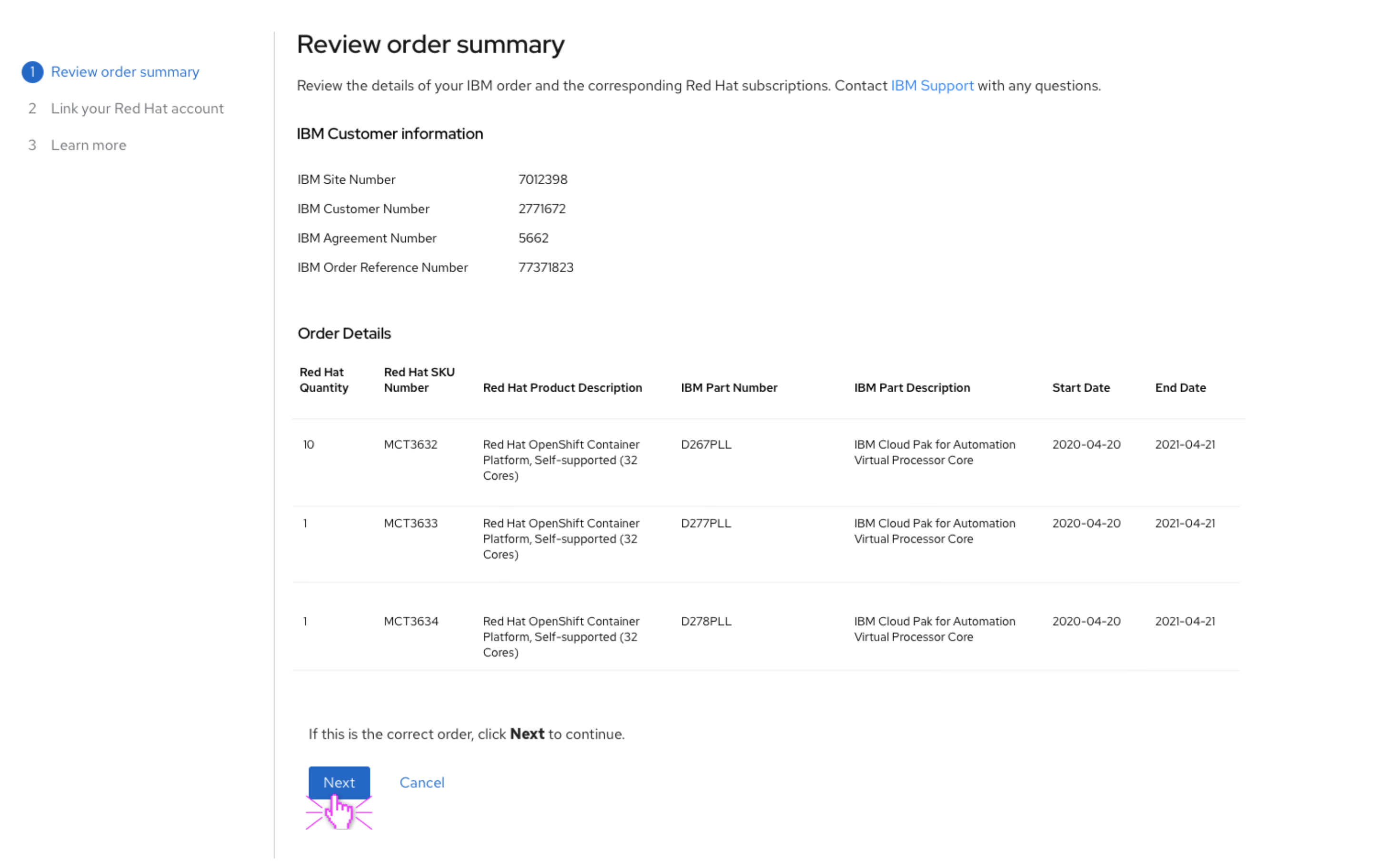**IBM Order Summary Screenshot**

This image showcases a screenshot of an IBM order summary on a clean white background. The focal point is the "Review Order Summary" title prominently displayed in bold black letters. Below the header is an instructional line in smaller text: "Review the details of your IBM order and the corresponding Red Hat subscriptions." Additionally, there's a clickable "IBM support" link highlighted in blue for contact purposes in case of questions.

The subsequent section is labeled "IBM Customer Information" and contains the following details:
- **IBM Site Number**: 7012398
- **IBM Customer Name**: 2771672
- **Customer Number**: 2771672
- **IBM Agreement Number**: 5662
- **IBM Order Reference Number**: 7737823

Following this, the "Order Details" section is presented, comprising seven columns with the headings:
1. Red Hat Quantity
2. Red Hat SKU Number
3. Red Hat Product Description
4. IBM Part Number
5. IBM Part Description
6. Start Date
7. End Date

The table lists three order lines with specific data:

1. **First Line**:
    - **Quantity**: 10 
    - **Red Hat SKU**: MCT3632
    - **Red Hat Product Description**: Red Hat OpenShift Container Platinum Self-Supported (32 COVES)
    - **IBM Part Number**: D257PLL
    - **IBM Part Description**: IBM Cloud Pak for Automation Virtual Processor Core
    - **Start Date**: 2022-04-20
    - **End Date**: 2023-04-21

2. **Second Line**:
    - **Quantity**: 1 
    - **Red Hat SKU**: MCT3633
    - **Red Hat Product Description**: Red Hat OpenShift Container Platform Self-Supported (32 cases)
    - **IBM Part Number**: D377PLL
    - **IBM Part Description**: IBM Cloud Pak for Automation Virtual Processor Core
    - **Start Date**: 2020-04-20
    - **End Date**: 2021-04-21

3. **Third Line**:
    - **Quantity**: 1 
    - **Red Hat SKU**: MCT3634
    - **Red Hat Product Description**: Red Hat OpenShift Container Platinum Self-Supported (32 cases)
    - **IBM Part Number**: D278PLL
    - **IBM Part Description**: IBM Cloud Pak for Automation Virtual Processor Core
    - **Start Date**: 2020-04-20
    - **End Date**: 2020-04-21

The section concludes with a prompt: "If this is the correct order, click Next to continue," accompanied by a blue "Next" button denoted by a pink finger pointing at it, or an option to cancel.